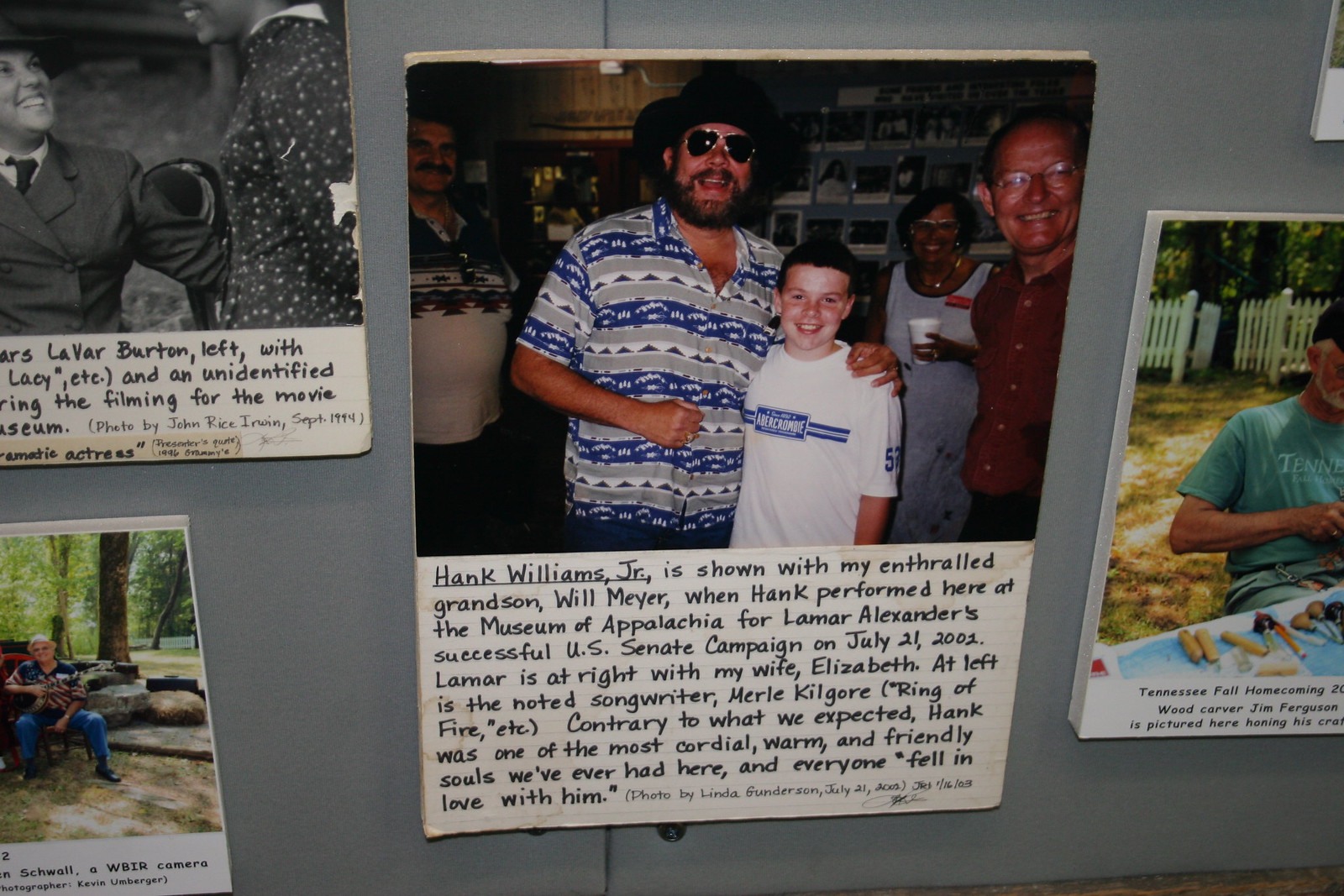This image consists of several photographs mounted on a gray wall, forming a nostalgic collage. The central photo depicts Hank Williams Jr., wearing a black brimmed hat, gold-rimmed sunglasses, and a striped gray, white, and navy shirt, with his arm around a smiling boy in a white T-shirt. Behind them are three other individuals: a black woman in a sleeveless white dress holding a white styrofoam cup and a smiling white man in a brown shirt with glasses and receding hairline. The caption below this main photo reads, "Hank Williams Jr. is shown with my enthralled grandson, Will Meyer, when Hank performed here at the Museum of Appalachia for Lamar Alexander's successful U.S. Senate campaign on July 21, 2002. Lamar is at right with my wife, Elizabeth; at left is noted songwriter Mary Kilgore (Ring of Fire, etc.). Contrary to what we expected, Hank was one of the most cordial, warm, and friendly souls we've ever had here. Everyone fell in love with him."

Flanking this central image are three more partially visible photos. In the upper left corner, a black-and-white photo shows a man in a suit and tie, smiling and arm around a woman in a black dress with a white collar and polka dots. Below this is a color photo of a man sitting on rocks in a forest, wearing blue jeans, a dark shirt, and a light-colored hat. The image on the far right depicts a man in a blue T-shirt at a white table with a blue cover, possibly with carrots on it, and a white picket fence and green-leaved tree in the background.